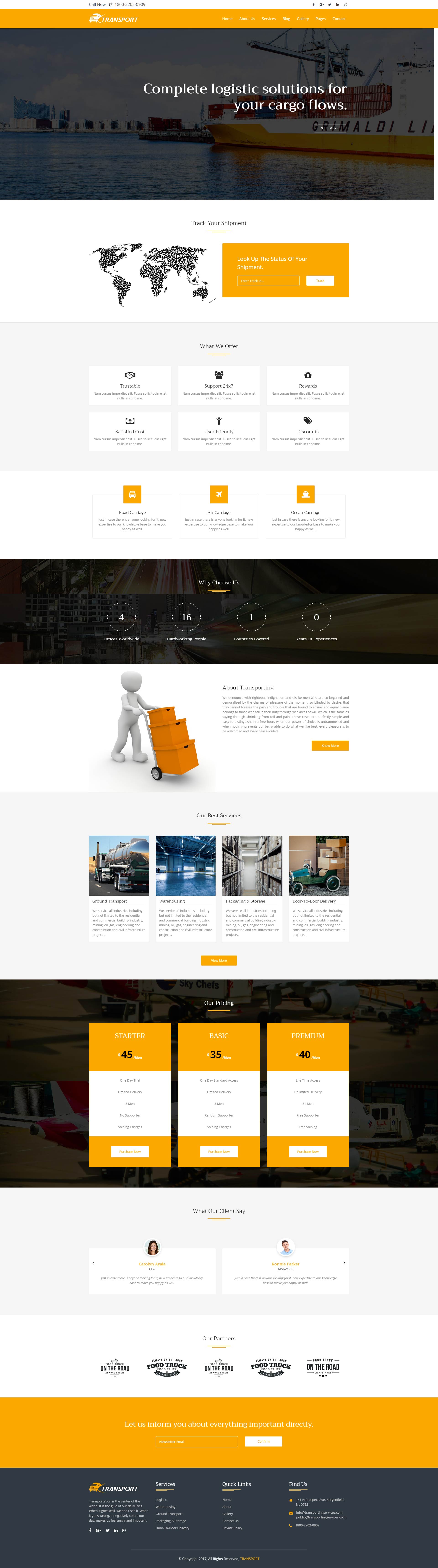This is a detailed image caption of a screenshot from a smartphone displaying the website for "Complete Logistics Solutions for Your Cargo Flows". The layout is structured into layers, featuring both white and light gray content sections separated by black borders. 

At the very top of the screen, a world map is displayed in a white section, highlighting land masses and waterways. Following this, there's a light gray section containing a grid of nine boxes, although the text within them is not legible. 

Subsequent to this, another white section appears, featuring three orange boxes. Below this, encased in a black border, are circles containing the numbers 4, 16, 1, and 0. 

Further down, a caricature of a person is depicted pushing three boxes on a dolly within another section. Below this, there are four images placed in a gray section; however, the specifics of these images remain unclear. 

Then, a black section features four distinct boxes displaying "4S", "3S", and "4.0" in the first, second, and last boxes respectively. This is followed by another gray section with what looks like two users' photos. 

At the bottom of the page, there is another white section containing advertisements, followed by an orange section, and finally, another black bordered section with additional info that is too small to be read clearly.